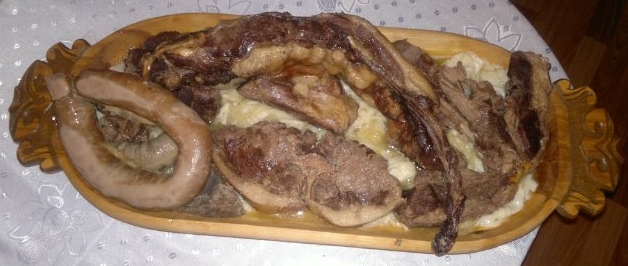The photograph showcases a lavish wooden serving tray with ornate, crown-like handles, placed on an intricately embroidered white tablecloth. The tablecloth features detailed silver flowers and dots, creating a subtle sheen against the dark wooden table visible underneath. The tray itself is oval-shaped and wide, holding an assortment of various meats, predominantly glazed and sauced. On the left side, there's a long, curled sausage, while the center hosts a sizable steak-like cut of meat. Towards the top, a piece resembling bacon or pork loin sprawls across the tray. Several other ambiguous cuts of meat occupy the remaining space, including a peculiar brown piece at the top that arches and tapers into a rounded point. Interspersed among the meats are hints of starchy vegetables, possibly mashed potatoes or a white, creamy substance, contributing to the overall hearty appearance of the meal.